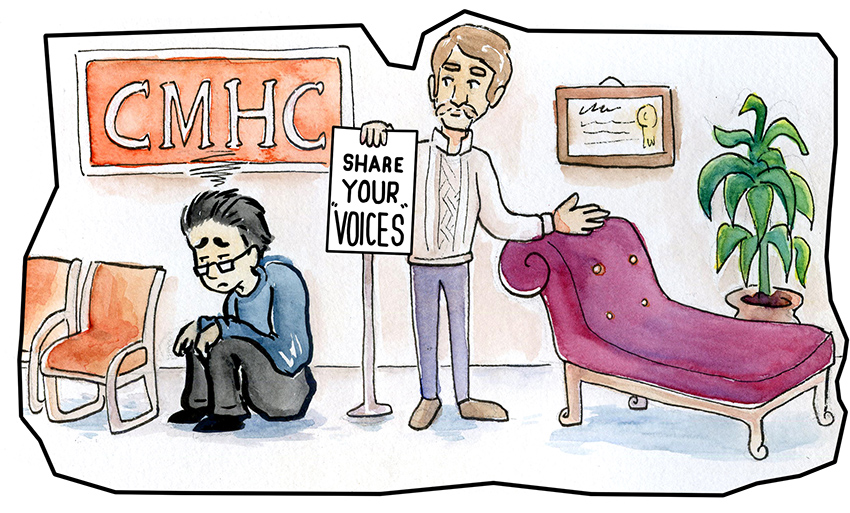This watercolor comic-style illustration depicts a scene inside a psychiatric or therapy clinic. On the left side, an orange sign with a black outline reading "CMHC" hangs above a row of matching orange waiting chairs. Below the sign, a person in a blue shirt, black pants, and glasses sits on the ground, looking noticeably depressed. 

To the right, a therapist with light brown hair, wearing a gray sweater, blue pants, and brown shoes, stands holding a sign that says "Share Your 'Voices.'" His other hand points towards a maroon lounge chair, typical of a therapist's office. The wall behind him features his degree or certification, and a tall plant stands beside the lounge chair, adding a touch of greenery to the scene.